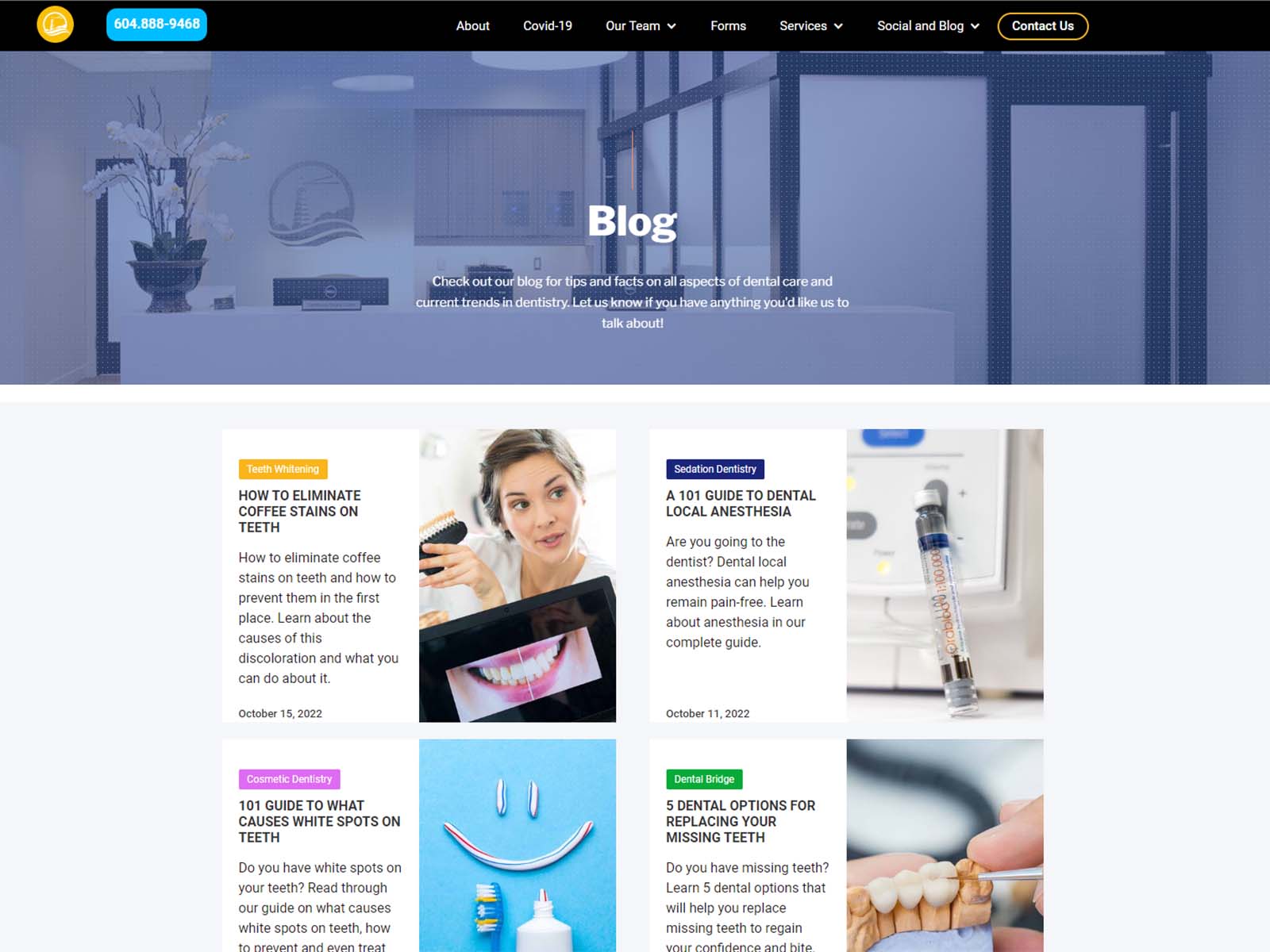This screenshot captures a blog focused on dental care. The top half showcases a user-friendly design, featuring a phone number prominently displayed within a blue oval in the upper left-hand corner, accompanied by a yellow circle adjacent to it. A sleek black bar runs along the top, hosting the website's menu options. Dominating this section is a large rectangular photograph depicting a modern dental office's check-in desk, with an overlay of white text stating "Blog" alongside an invitation to "Check out our blog for tips and facts on all aspects of dental care."

In the bottom half of the webpage, four distinct squares each highlight a different blog topic with corresponding visuals and textual descriptions. The first square, accentuated with a yellow bar, is dedicated to "Teeth Whitening" and features an image of a smiling woman. Adjacent to it, the second square focuses on "Sedation Dentistry," marked by a blue bar and a photograph showing a vial of medicine and medical equipment. The layout is visually engaging and informative, guiding readers through various aspects of dental health.